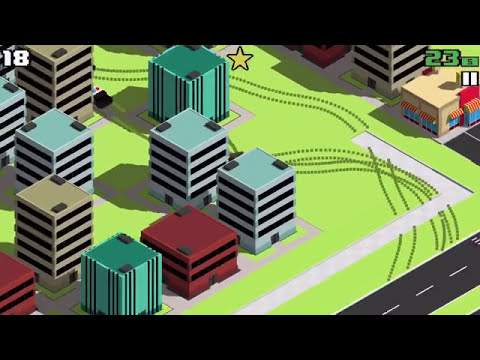The image is a screenshot from what appears to be a simulation or city-building mobile game, featuring a cityscape with a distinct, somewhat pixelated graphic style akin to The Sims or SimCity. Dominated by a green grassy expanse, the scene showcases various buildings: light blue, green, cream-colored, and dark red, with a central cluster of around seven to eight structures. Notably, in the upper center area, there's a yellow star, while the top left corner displays a white "18" logo. In the top right, a green "23" is visible, followed by a green "5" next to it. Among the buildings, one resembles a store or fast food chain, recognizable by its cream facade, blue windows, and red-yellow striped canopies. This building also features a parking lot. The game-like environment includes tire marks scattered across the grassy area, suggesting vehicle movement, and a black-and-white street on the bottom left. A partly shadowed police car with noticeable red and blue lights is also distinguishable in the lower parts of the image.